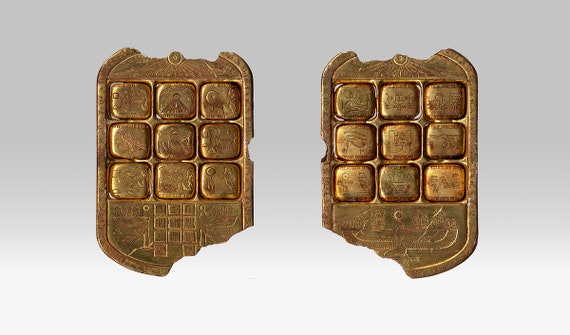The image depicts two ancient artifacts that appear to be tablets or possibly items used for trade, likely of cultural or historical significance. Both artifacts have a rounded square shape, with the top parts and bottom intersections broken off. Each artifact features a grid-like pattern composed of nine golden squares or nodules, arranged in a three-by-three grid on their surfaces. On the left artifact, this grid is prominently displayed at both the top and the bottom, with a segment of the bottom right corner missing or broken. The artifact on the right also showcases this grid pattern, with its bottom left corner visibly damaged. Additionally, the right artifact appears to have an imprint resembling an eagle or a bird at the very bottom, suggesting a possible insignia or seal. These elements, along with the worn and ancient appearance, evoke a sense of the artifacts being relics from a civilization similar to the Mayan or Aztec.